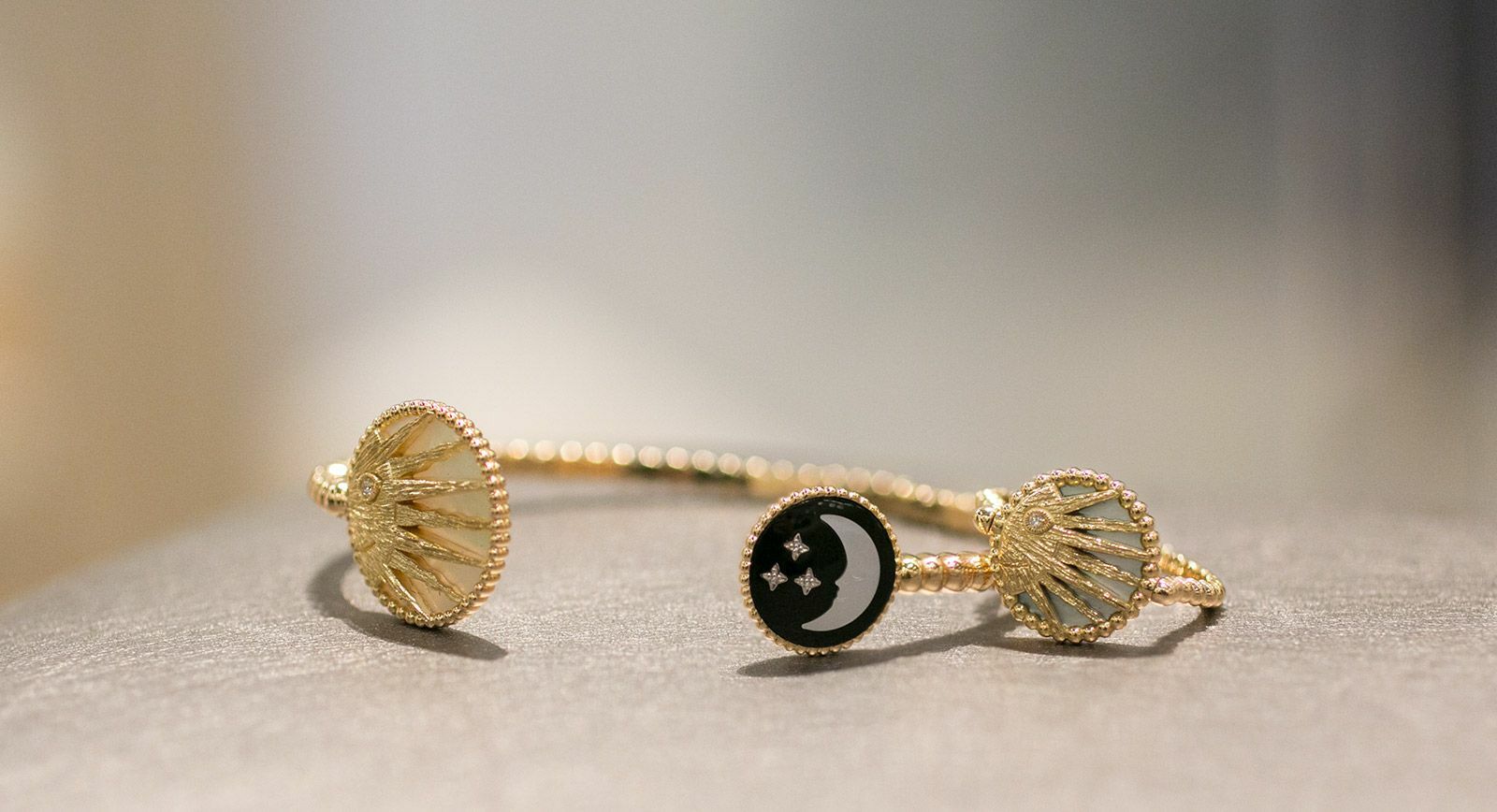The image showcases an intricately designed, elaborate golden bracelet set against a smooth, blurred gray background. The bracelet features a series of rounded, gold ridges or bulbs that run along its surface, enhancing its luxurious appeal. On the left side, a circular gold emblem with a prominent, ornate crown design, detailed with seven pointy spikes and a pearly white background, adds a regal touch. Towards the right, a striking black circular segment stands out, adorned with a white crescent moon and three diamond-studded stars, set within a gold border. Near this black and gold motif, another similar emblem is visible, suggesting a paired design theme within the bracelet. The close-up nature of the image highlights the craftsmanship and brilliance of the bracelet, emphasizing its shiny, elaborate, and potentially expensive appearance.